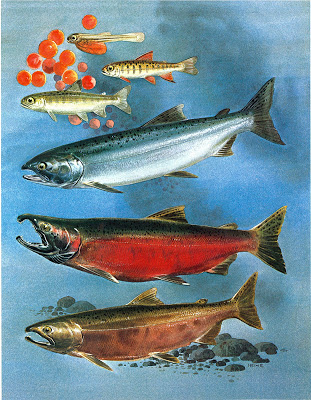This illustration features six distinct fish swimming to the left against a vividly layered blue background that transitions from teal to pale blue and dark blue. At the top, three smaller fish are slightly askew but aligned vertically, clustered around red bubbles, which could represent fish eggs or air bubbles. These top fish exhibit a mix of orangish and greenish-gray hues, with stark white bellies and prominent black pupils in their eyes. Beneath these smaller fish, there are three larger fish, each uniquely colored and patterned. The fourth fish from the top is primarily blue with black specks and a light belly. The fifth fish showcases a striking combination of red and black, possibly hinting at a salmon species. The bottom-most fish displays a pink hue with green and black speckles on its upper part. In the foreground near the bottom of the image, various-sized gray rocks add to the underwater scenery. The entire composition, with its detailed portrayal of fish and a textured aquatic background, presents a lively and intricate underwater tableau.